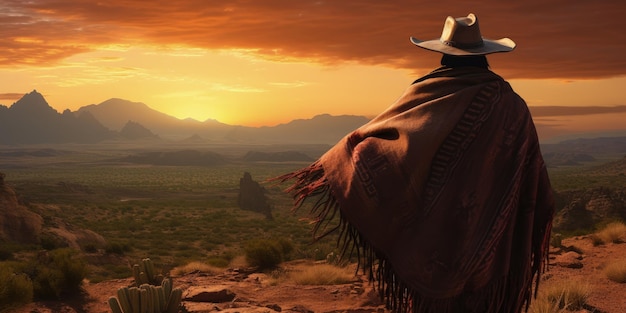In this color illustration of a desert landscape at sunset, a lone cowboy stands prominently in the foreground on the right-hand side. Clad in a large, broad-brimmed hat and a long, fringed poncho that drapes over his shoulders and flutters in the breeze, he gazes towards a vast grassy plain that extends to the horizon. The ground beneath him is a reddish-brown dirt, interspersed with cacti, dried bushes, and tumbleweeds. To the left of the cowboy, a prominent rock formation juts upward. In the distance, a row of purple mountains with a mixture of peaked and rolling hills contrasts against the glowing gold and yellow hues of the setting sun. The upper part of the sky is darkening, filled with horizontal clouds tinged in dark orange due to the sunset. The entire scene evokes the mystique and rugged beauty of the Old Wild West.